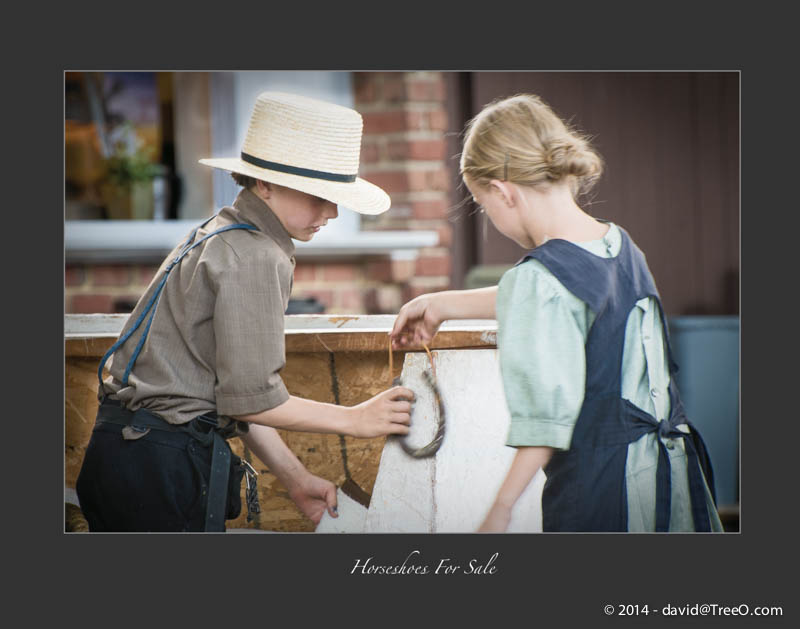The image is a color photograph set against a wide gray border with white text beneath it that reads "Horseshoes for Sale" in cursive. In the lower right corner, there is a copyright notice from 2014. The photograph features two young children dressed in traditional Amish-style clothing. The boy on the left wears a broad-brimmed straw hat, brown top, black pants, and suspenders, while the girl on the right has dirty blonde hair tied back and wears a blue dress with a smock-like apron. Both children are holding onto a horseshoe attached to a string, and they stand in front of a red brick wall with a window framed in white visible in the background.